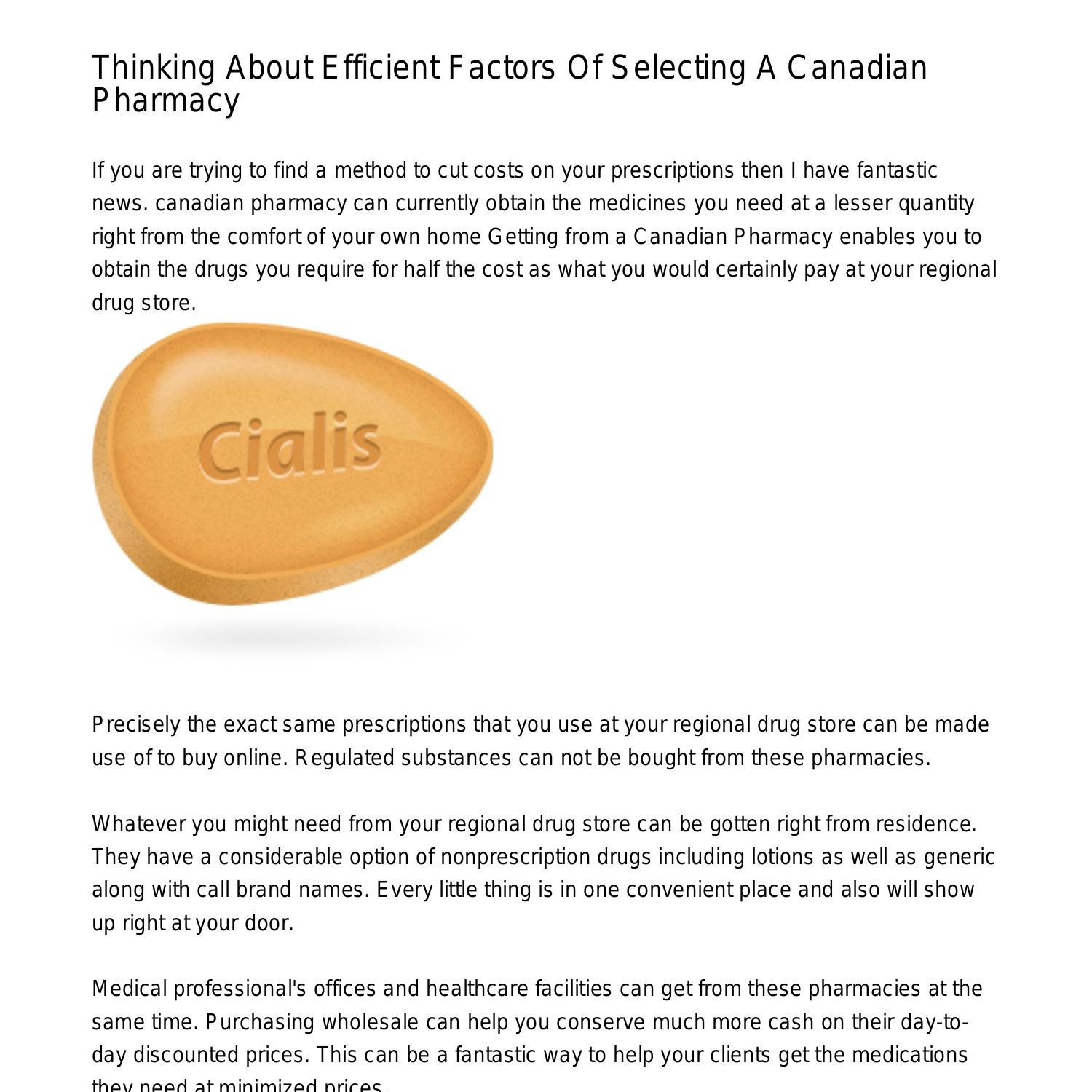This screenshot captures a detailed information page about various Canadian pharmacies. At the top of the image, a bold title reads, "Thinking About Efficient Factors of Selecting a Canadian Pharmacy." Below the title is a well-composed paragraph highlighting the cost-saving benefits of using Canadian pharmacies, suggesting that a Canadian pharmacy can offer prescriptions at a considerable discount compared to local drug stores. The text emphasizes the convenience of obtaining medications from the comfort of one's home and at a lower price.

Following this textual information, there is a prominent, zoomed-in image of a pill or vitamin, which appears to be a computer-generated graphic rather than a photograph. The pill is yellow, teardrop-shaped, and oriented on its side with the label "Cialis."

Beneath the image, the page continues with three additional short paragraphs. These paragraphs convey that the prescriptions available at local drug stores can also be purchased online from Canadian pharmacies. It is noted that regulated substances are not available. The content highlights the extensive selection of over-the-counter medications, including both generic and brand-name products, all available in one convenient place and delivered directly to the door. The paragraphs also mention that medical professional offices and healthcare facilities can place bulk orders, providing an opportunity to save even more on everyday discount rates, thus benefiting their patients with reduced medication costs.

This descriptive account provides readers with a thorough understanding of the image's content and message, illustrating the potential financial advantages and convenience offered by Canadian pharmacies.